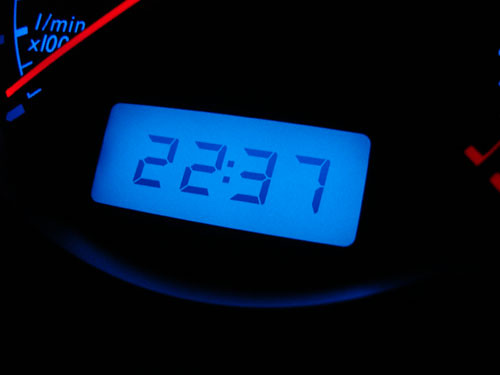The image portrays a blue-illuminated digital display showing the time in a 24-hour format, reading 22:37. The background is predominantly dark, suggesting the photograph was taken at night. To the top left corner of the image, a portion of a circular odometer is visible, indicating that this scene is likely from the dashboard of a vehicle. The odometer segment displays a red needle and numbered markings, with some increments labeled as "x100." The overall dim lighting and specific details contribute to a nighttime setting inside a vehicle.